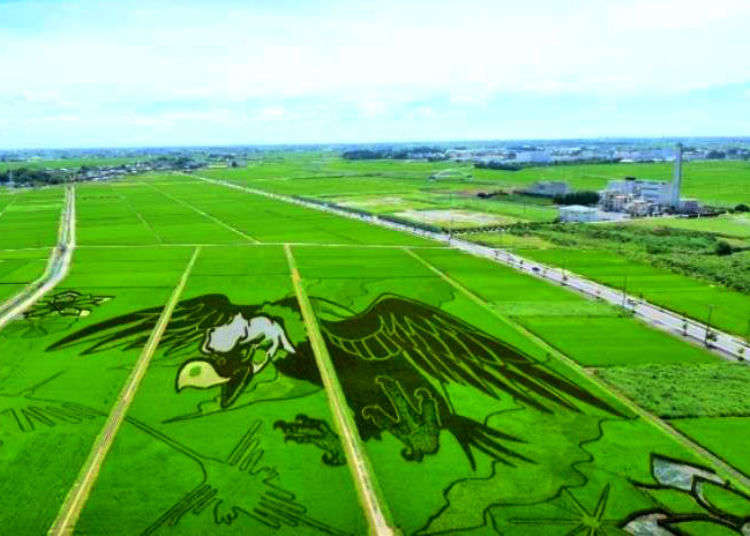This aerial image showcases an intricately designed field in what appears to be the Midwestern United States, possibly Iowa, created either by planting crops in distinct patterns or mowing the grass into shapes. The focal point of the landscape is a massive, cartoony bird—perhaps a phoenix, eagle, or vulture—with a striking white head, a yellow beak, and eyes looking downward as if it's about to land or attack. Its claws are extended toward the viewer, giving a dramatic effect. The bird's wings are pulled back, further enhancing the lifelike yet stylized representation.

The bird is positioned in the lower center of the image, surrounded by various other designs, including large flowers carved into the field and smaller bird-like figures below it. On the left side of the image is a white farm or factory with a small, tall smokestack. The farmland extends above this structure, meeting with roads that wind through the field, providing a sense of scale as they accommodate cars.

Two main roads are visible: one begins at the center left and curves towards the right, while another runs along the right side of the bird. In the distant background, obscured by the vast expanse of the designed farmland, a cityscape emerges, adding depth to the image. The green fields are punctuated by blue skies above, highlighting the contrast between the natural landscape and human-made artistry. Overall, this image captures a remarkable blend of agricultural ingenuity and artistic expression.